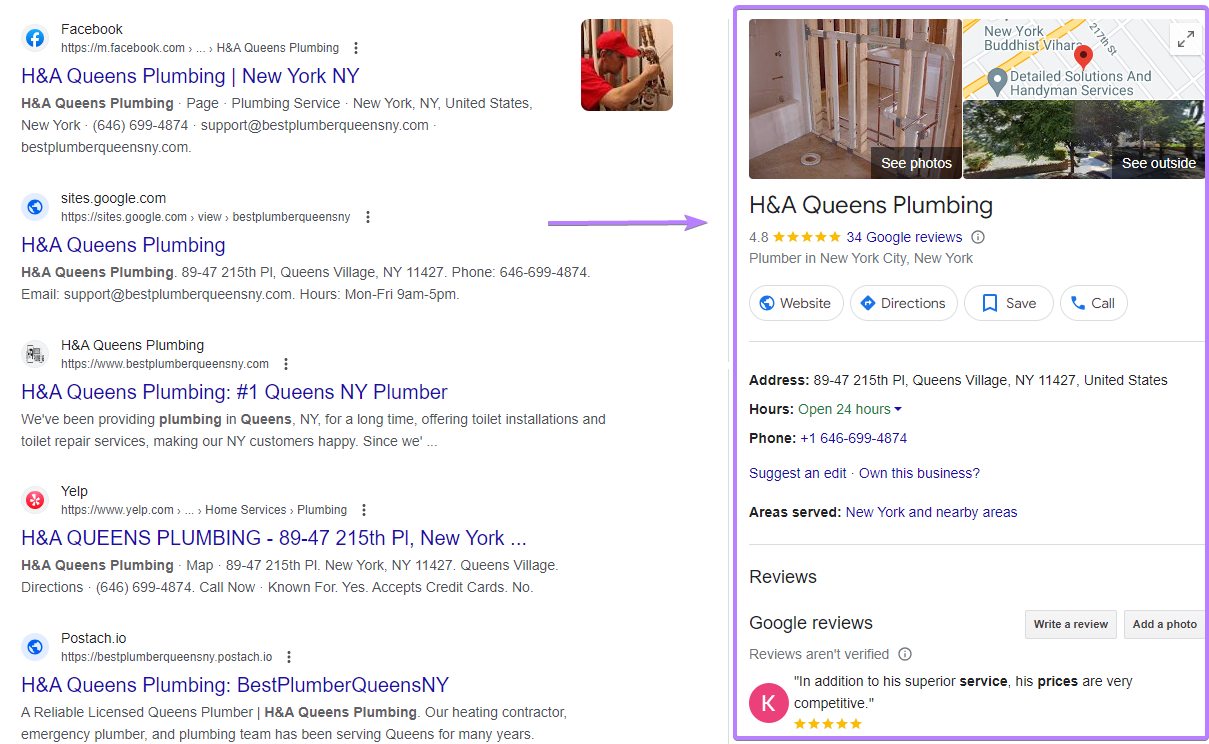This is an image of a search results web page, distinguished by its dark purple text. The search field is absent from view. On the left-hand side, there are five outlined results. The top result is associated with a Facebook icon, labeled "Facebook."

The second result is somewhat unclear, with text in black ink that's difficult to read. 

The third entry focuses on "H.A. Queens Plumbing, New York, NY" and is highlighted with purple ink. It contains detailed contact information including a phone number, a support email, and the website "Best Plumbing, Queens, New York dot com," all in tiny black ink. This is the only search result that features an image—depicting a white plumber in a red cap and red shirt, seemingly engaged in plumbing work.

The fourth result includes a globe icon and the URL "sites.google.com." Below that, the text is in black and somewhat illegible, followed by "H.A. Queens Plumbing" written in purple. Detailed information about H.A. Queens Plumbing is provided in a small black font. This entry uniquely features a purple arrow pointing to the right, detailing more about H.A. Queens Plumbing, including an image of copper pipes inside a house. To its right is a map showing the location of H.A. Queens Plumbing, accompanied by a photo labeled "see curbside." Adjacent to this map, the caption "see photos" suggests additional images encompassing the premise's plumbing. In black ink, the entry states "H.A. Queens Plumbing," a 4.8 rating, asserted by five gold stars, and supported by 34 Google reviews. Additionally, the status "open 24 hours" is mentioned, along with an address, contact number, website links, directions, saving options, and a call button. Further down, it mentions "areas served in New York and nearby areas." Reviews are indicated in black ink, followed by grey buttons for writing a review and adding a photo. The notice "reviews aren't verified" appears in tiny grey font.

The fifth and final result features "H.A. Queens Plumbing" again with an indistinct grey icon to the left. Labels such as "number one Queens New York Plumber" appear in purple, coupled with additional information. Below this, a rose-colored Yelp icon is followed by the text "Yelp" in black. The address "8947 215th Place, New York" is highlighted in purple, with further information listed below. The subsequent item has a globe icon and the term "POSTACH" beside it, and once again, features "H.A. Queens Plumbing" in purple, concluding with more plumbing company data underneath.